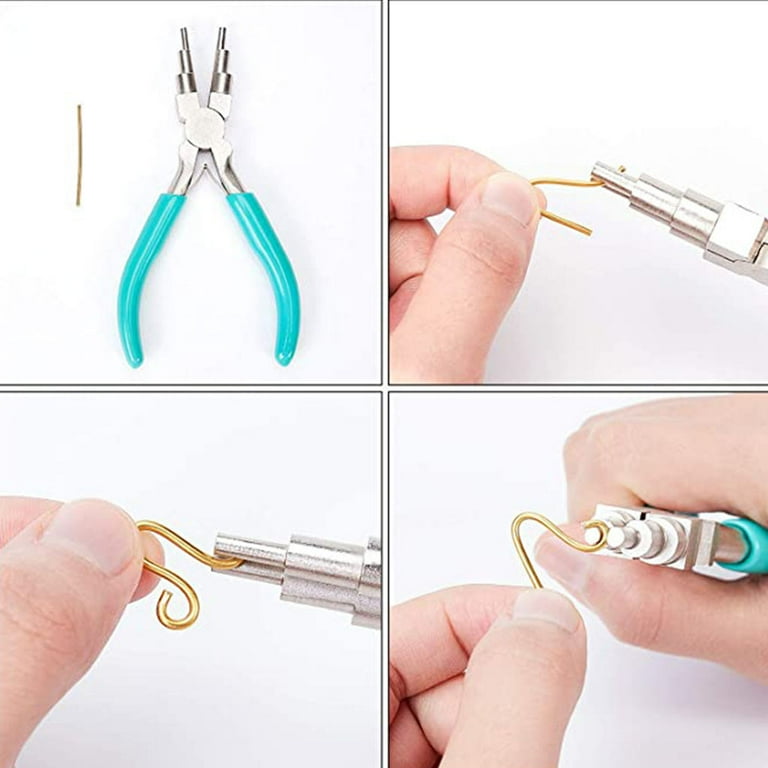This color photograph is divided into four equal sections, each featuring a close-up view of a hand-held tool being used to bend a gold-colored copper wire. In the top left section, a tool resembling pliers with turquoise handles lies next to a straight piece of gold wire. The top right section shows a Caucasian hand holding the tool as it starts to curve the wire. In the bottom left section, there's a more detailed close-up of the further curved wire, revealing intricate bends. Finally, the bottom right section captures a different angle of the tool at work, with the left hand holding the wire and the right hand operating the tool to complete the bending process. The background in all images is white, emphasizing the tool and its function, perhaps for making jewelry.